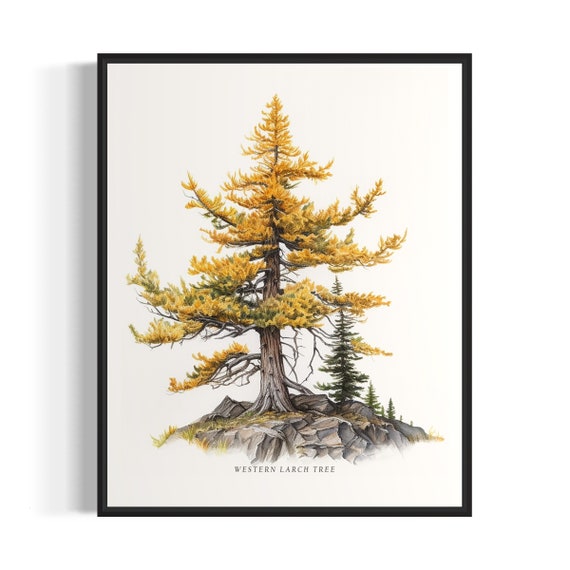The image is a framed illustration of a tall Western Larch tree with the label "Western Larch Tree" written in slight italic capital letters beneath it. The illustration is on a white background and encased in a black frame with a noticeable shadow to the left, suggesting it may be hanging on a wall. The tree is depicted with long, sturdy branches extending outward and adorned with yellowish-gold leaves, indicating a fall setting. It is growing atop a rocky terrain, with some needles scattered on the boulders below. The bark is a lighter brown or grayish brown. In the background, there are several successively smaller, spindly evergreen trees, which remain green, contrasting with the autumnal colors of the Western Larch.